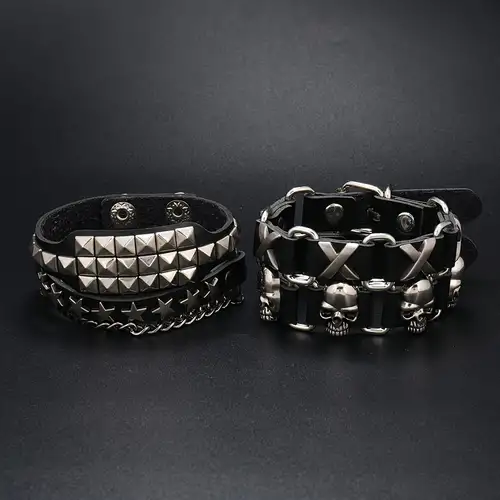The image features a black and grayish background showcasing two distinct belts, often associated with goth or emo fashion, perhaps reminiscent of items found at Hot Topic. The belt on the left side is predominantly black and adorned with intricate designs. It features small, silver pyramid studs arranged in a detailed pattern on the upper part, and a series of silver stars circling around its black buckle at the bottom. On the right side, there is another black belt that stands out with a combination of metallic embellishments. This belt is elaborately decorated with alternating metal skulls and X-shaped figures, creating an edgy, repetitive pattern. Both belts display a striking contrast of black and silver elements, set against a dark backdrop, emphasizing their bold, youthful style.